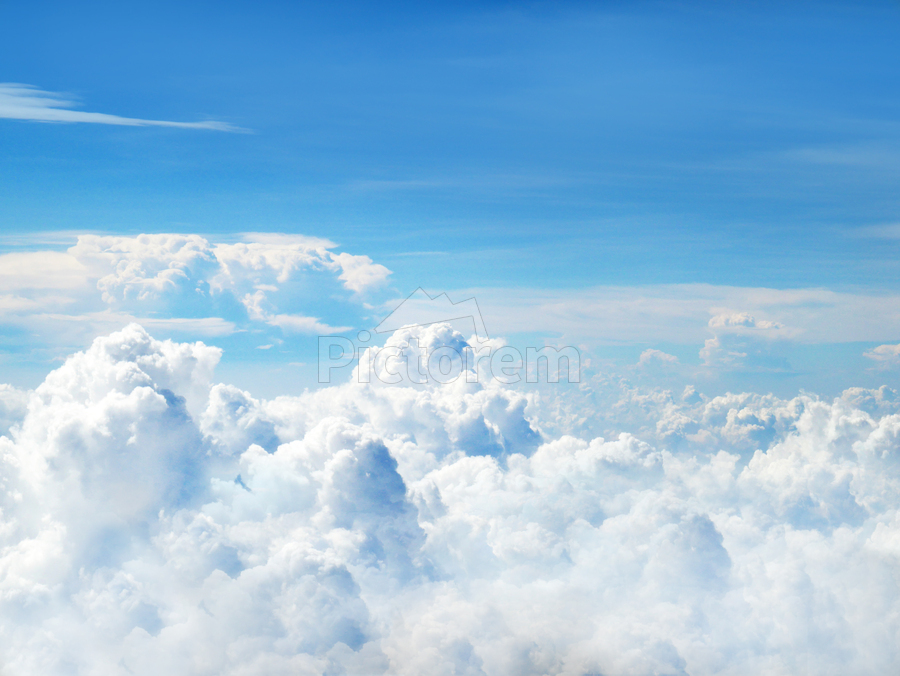The image depicts a serene aerial view, seemingly taken from an airplane at a high altitude, capturing a tranquil scene above the clouds. At the bottom, a vast expanse of fluffy, cotton-like clouds stretches across the horizon, meshing together in shades of light gray and white, with some areas outlined faintly in dark blue. These clouds exhibit significant texture and dark shadows, likely where they curve away from the sunlight. Above this cloud layer, a clear blue sky emerges, transitioning from a lighter blue at the center to a darker shade towards the top. A singular, thin white line streaks across the top left corner of the sky. The photograph is watermarked in the center with the text "pictorem," accompanied by a small mountain icon. The overall scene is simple yet captivating, evoking a sense of calm as if one is standing on the clouds and gazing into the infinite sky.